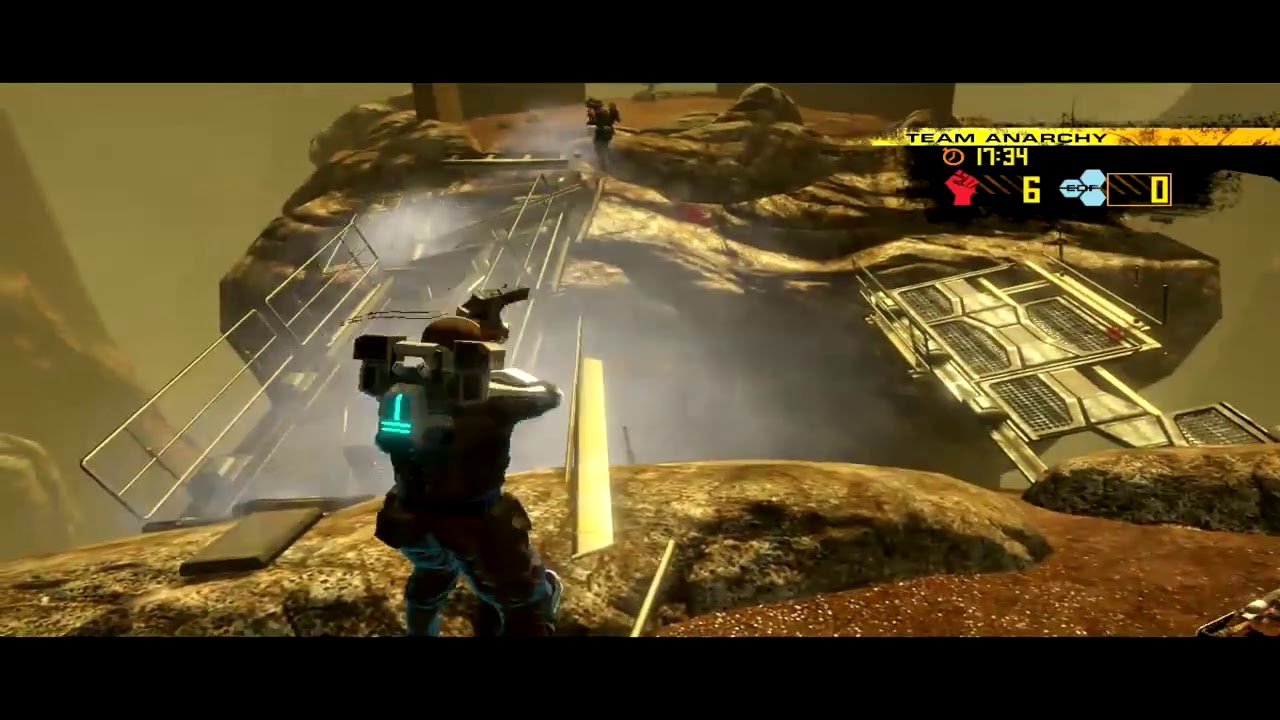The screenshot depicts a scene from a video game set on a rocky, outer space-like red planet, possibly Mars. In the foreground on the left, a person in a military-type space suit with a glowing upside-down T-shaped blue backpack is holding a weapon pointed across a ravine. On the other side of the ravine, another similarly dressed character faces the first person. Two metallic bridges flank this area, appearing broken or incomplete. To the top right, a white banner reads "Team Anarchy," below which a clock displays "17:34." Additionally, there is a red fist icon accompanied by the number 6, and a 0 nearby, likely indicating a score. The scene is outdoors and gives a sense of rugged, alien terrain.